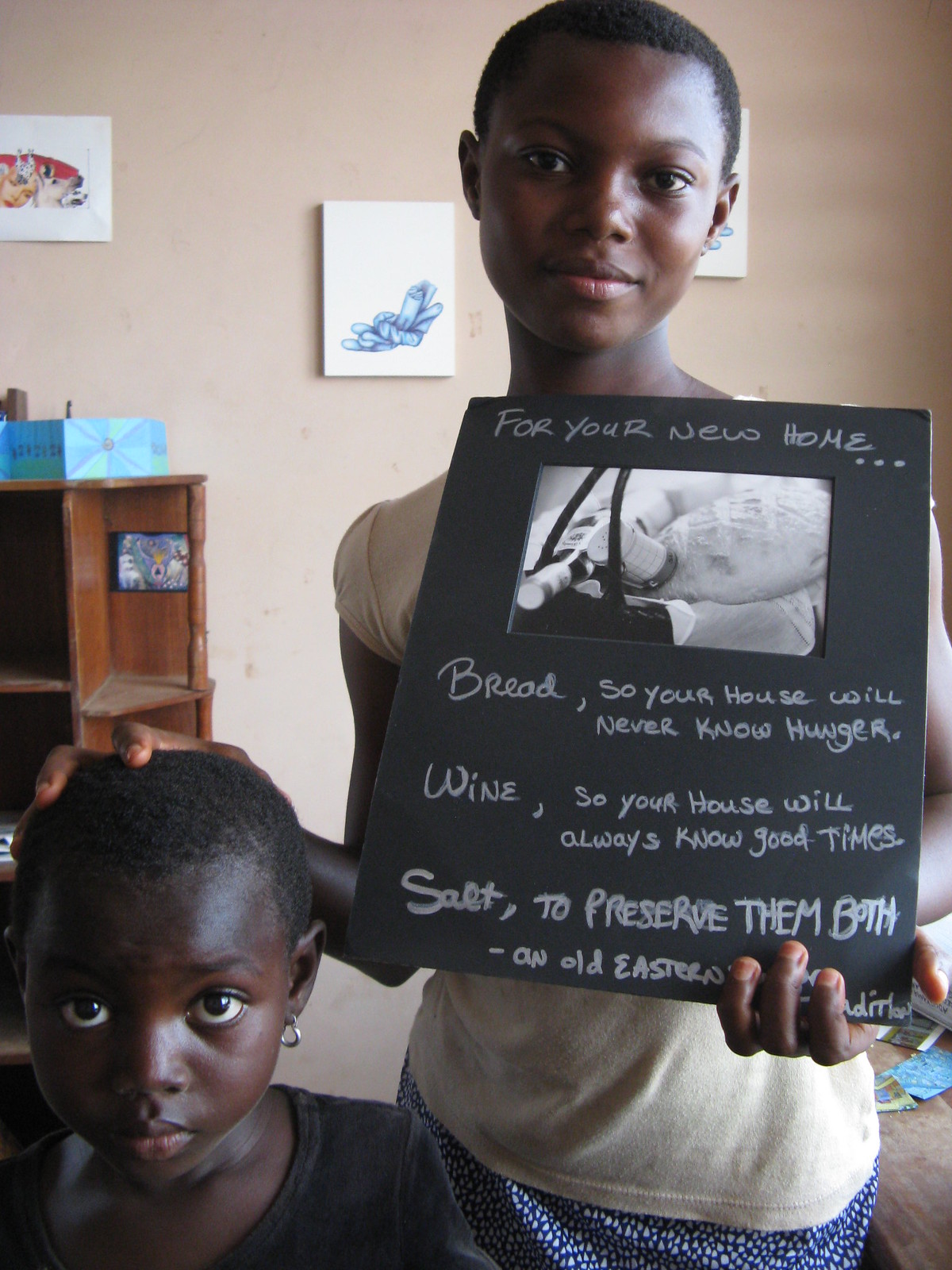In this image, a joyful African mother and her young child pose together, both with short hair and bright smiles. The mother, dressed in a cream-colored short-sleeved shirt and blue pants with small white dots, gently rests her right hand on the child’s head. The child, wearing a black shirt and an earring, gazes directly at the camera while being held.

The mother holds a black sign prominently in front of her, bearing an endearing message for a new home. The sign reads: "For your new home, bread so your house will never know hunger, wine so your house will always know good times, salt to preserve them both," ending with an obscured piece of text likely referring to an old Eastern tradition.

They are standing in a cozy living room with cream-colored walls adorned with various artworks. Behind them, there's a notable crystal depiction, an entertainment center showcasing African art, and several smaller pieces, including a striking 6x6 framed piece and a blue postcard-like art piece on a shelf. The warm backdrop and heartfelt sign create a scene that exudes love, culture, and the promise of a cherished home.